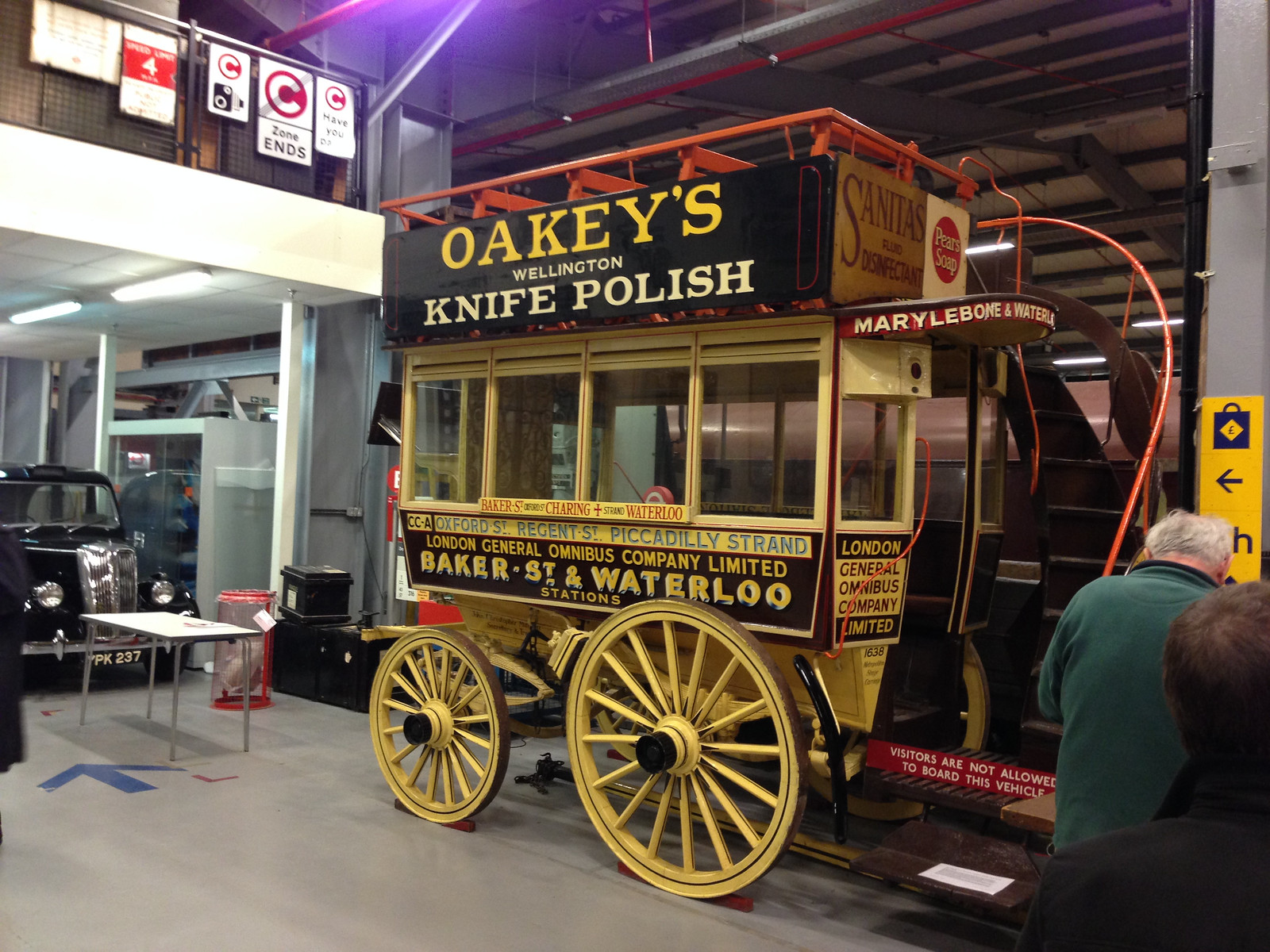This indoor photograph captures a meticulously detailed display of a historic yellow-tan Omnibus carriage, prominently situated within what appears to be a warehouse or museum. The warehouse features visible beams and rafters and includes a second-floor balcony on the left side with five signs hanging from its fence, including a notable red and white sign and three signs with a 'C' in a red circle, centered by a "Zone Ends" message. Beneath the balcony sits an old black car, possibly from the 1930s or 1940s, with a readable license plate "PK 237". 

Ahead of the car lies a folding table, some shelves, and a blue arrow painted on the concrete floor. The Omnibus wagon draws particular attention with intricate detailing: it has disproportionate wheels, with the front larger than the back, and hosts an open seating area on top featuring orange benches. Various signs adorn its body, with the largest on the side advertising "Oakey's Wellington Knife Polish" and additional signage proclaiming "Sanitas Disinfectant" and "Pears Soap" on the front. Windows surround the carriage, with location names around them, including "Baker Street,” “Charing Waterloo,” “CCA Oxford Street,” "Regent Street,” “Piccadilly Strand,” and “London General Omnibus Company Limited.” 

Above the entrance, the awning displays "Marylebone and Waterloo." Adjacent to the entrance is a staircase with an orange railing paired with a red sign warning visitors not to board the vehicle. The scene includes a white-haired Caucasian male in a green sweater with his back to the camera and an indistinct figure with dark hair and a dark sweater. Above their heads is a yellow sign marked with a suitcase and a left-pointing arrow, solidifying the vehicular display's immersive atmosphere.